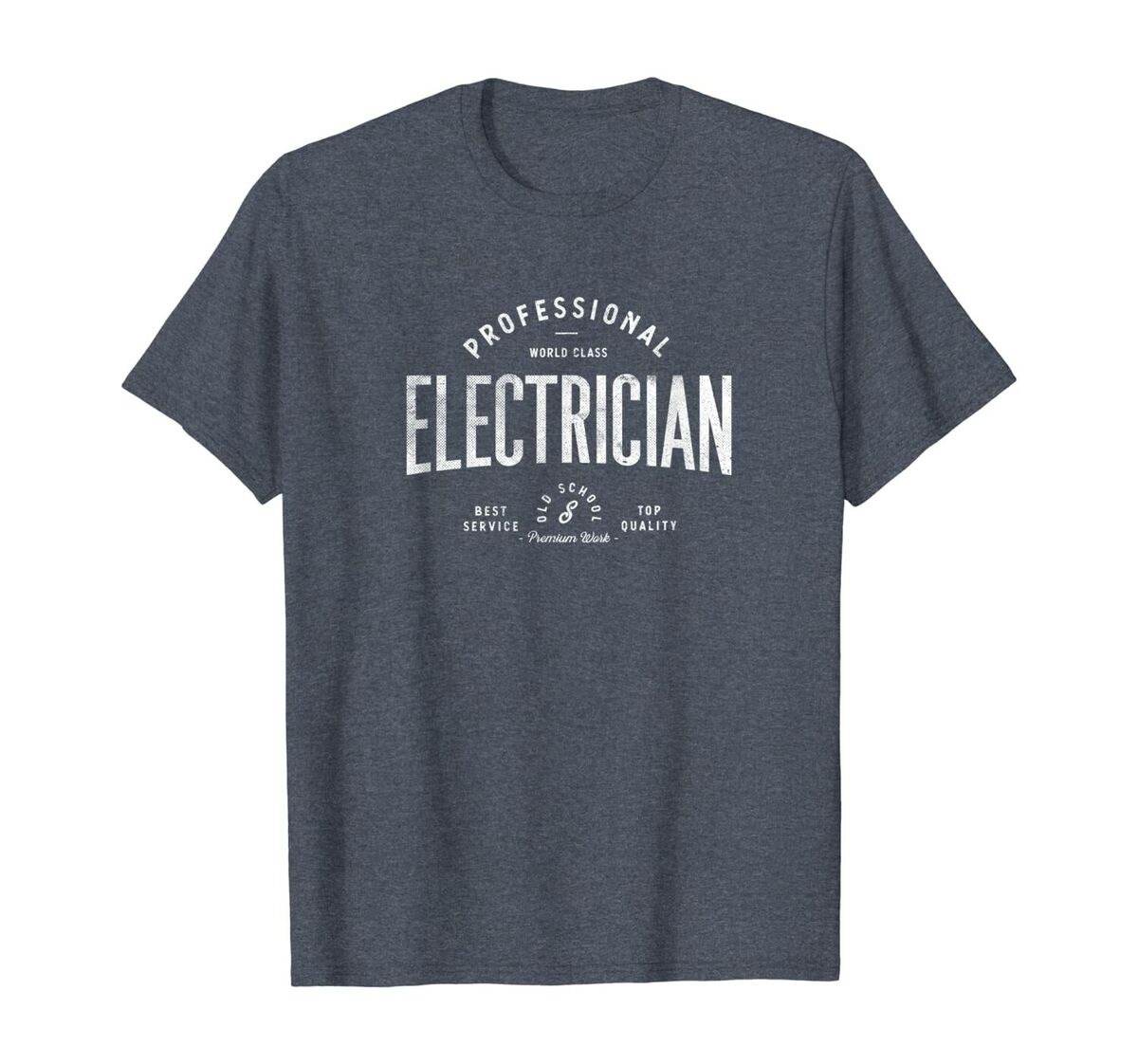The image depicts a dark gray (sometimes perceived as black or blue) t-shirt adorned with multiple inscriptions in white, uppercase text. At the top, curving around a circle, the word "PROFESSIONAL" is prominently displayed. Just below, a smaller curving text reads "WORLD CLASS." The largest text on the shirt, "ELECTRICIAN," is centrally located with a subtle inward curve at the bottom. Surrounding this are additional phrases such as "BEST SERVICE" to the left and "TOP QUALITY" to the right of "OLD SCHOOL," which is positioned below "ELECTRICIAN" with a decorative 'S' inside a circle. Lastly, "PREMIUM WORK" is written below the circular design. The shirt lacks a visible collar tag, contributing to its stock image appearance.